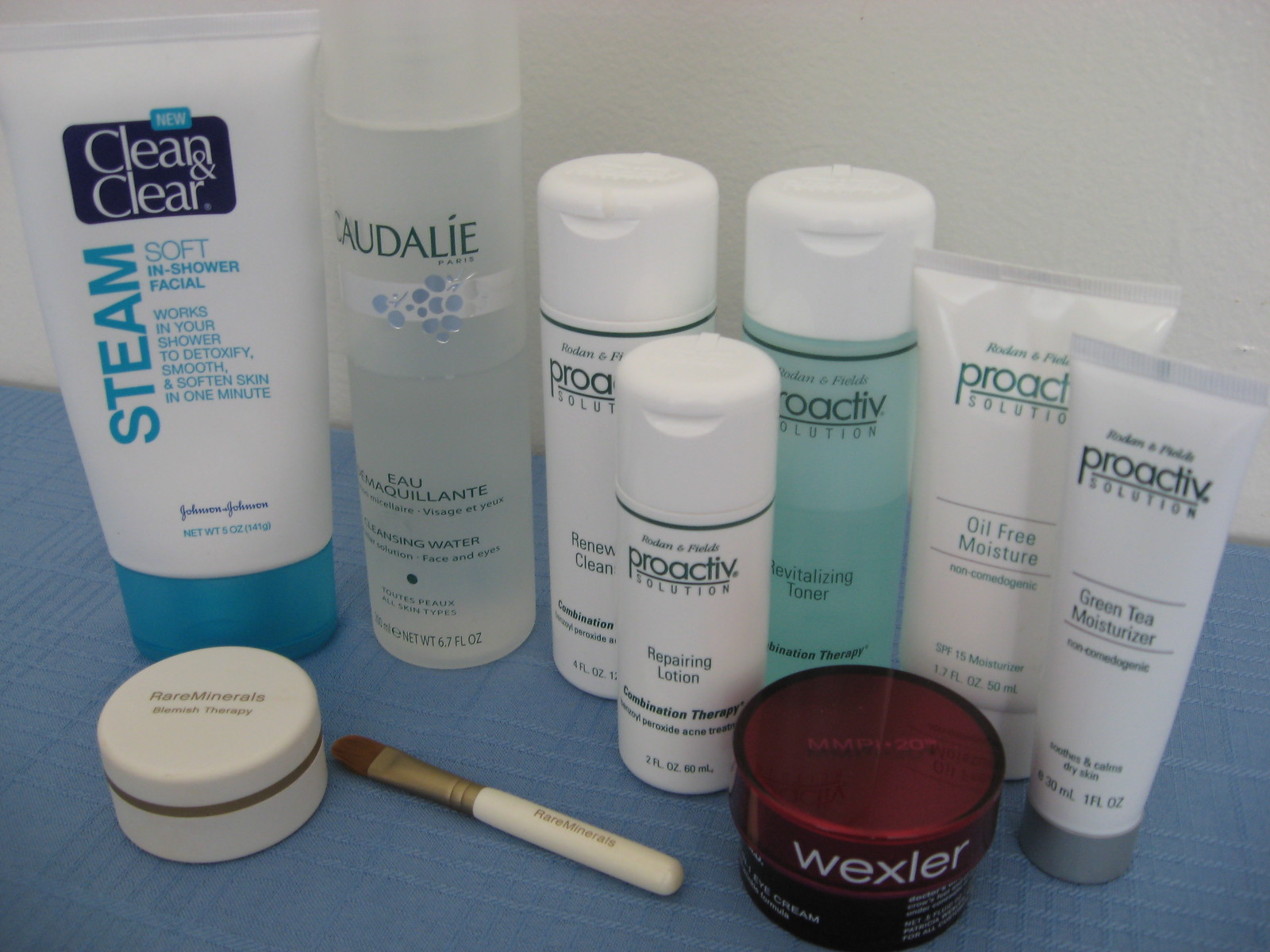The photograph presents an extensive and neatly arranged collection of facial care products spread across a blue countertop. Starting from the left, there is a white tube with a blue cap labeled "Steam Soft In-Shower Facial," which claims to detoxify, smooth, and soften the skin in just one minute when used in the shower. Adjacent to it is a small red canister labeled "Rare Minerals, Blemish Therapy," accompanied by a small applicator brush. Next to these items, there is a tall, clear bottle filled halfway with a French-labeled solution.

Moving rightward, the selection features a variety of Proactiv products. The first is a bottle labeled "Renew Cleanser," followed by another labeled "Repairing Lotion." There is also a more transparent, green-tinged bottle marked "Revitalizing Toner." Further along, there are two tubes: one labeled "Oil-Free Moisture" and the other "Green Tea Moisturizer." Finally, the collection concludes with a dark red burgundy canister with a lid that reads "Wexler." The organized display showcases a diverse range of skincare solutions, all neatly aligned on the vibrant blue surface.